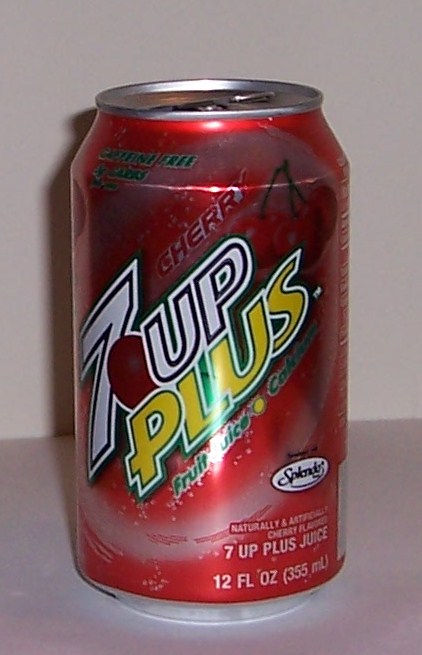This detailed photograph captures a red and pink can of Cherry 7-Up Plus soda, prominently featuring the Cherry 7-Up Plus logo in white and yellow writing. The can sits on a white tabletop and appears to be opened, as suggested by the visible opening at the top. To the right of the main lettering, there are vibrant images of three cherries. At the top left corner, in green letters, it reads "caffeine-free." Towards the bottom of the can, it notes "7-Up Plus juice" and "12 fluid ounces (355 milliliters)" in white text against the red backdrop. A distinctive white circle bearing the Splenda logo is visible near the bottom right section of the can. The overall layout includes various text angles and colors—gold, white, and black against the silver and red background—creating a visually dynamic design.